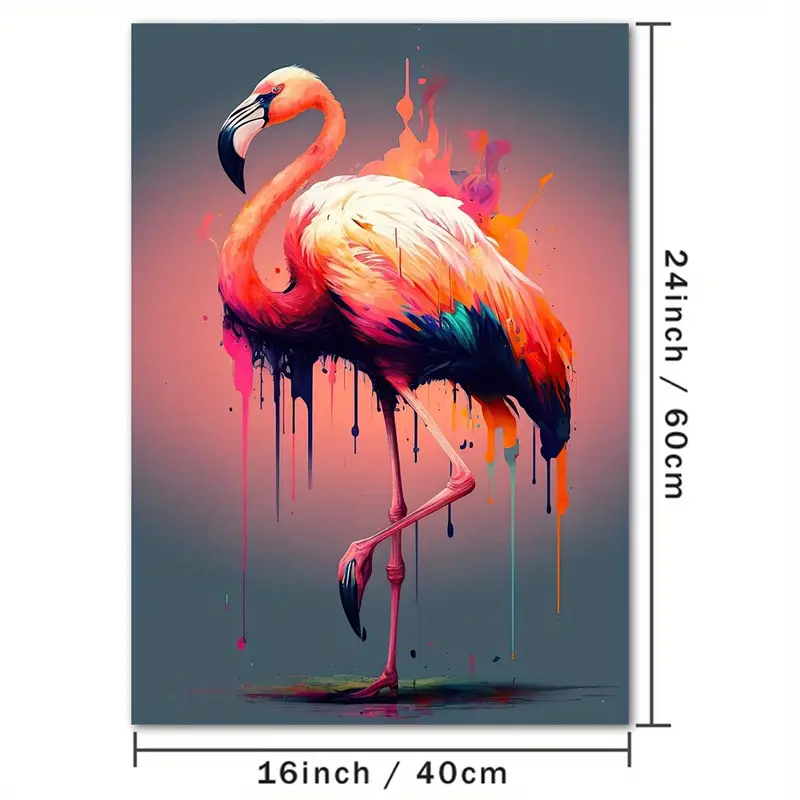This painting, measuring 24 inches (60 centimeters) in height and 16 inches (40 centimeters) in width, features a striking depiction of a swan. Set against a richly dark blue background with a prominent pink circle at its center, the scene exudes a dramatic and surreal atmosphere. The dark blue extends along the bottom of the painting, merging into a bluish-dark gray hue, creating a grounding effect. The swan itself is an artistic tour de force, its body rendered in various vibrant colors. The underbody of the bird merges seamlessly with the dark blue background, extending downward in a cascade of drips, as if the paint itself is melting off the canvas. The swan's elegant neck is painted a vivid pink, making a stark contrast to its softly light yellow back. In a dynamic finishing touch, the artist has splattered paint across the canvas, with each color running and dripping, creating an illusion that the painting is continuously in motion and adding a layer of spontaneity and excitement to the piece.